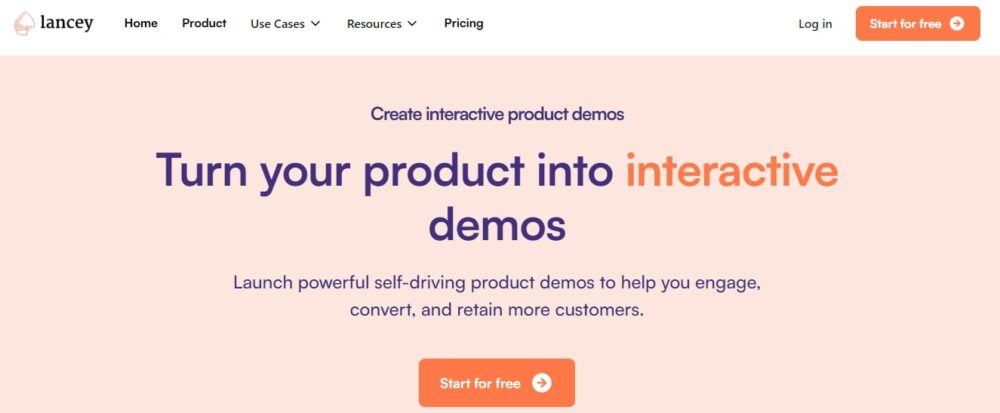This image is a screenshot of a landing page from a website called "Lancey." The website's name, "Lancey," is prominently displayed in the top left corner in sleek, black, lowercase letters. Adjacent to the site name is a horizontal navigation bar featuring links labeled: Home, Product, Use Cases, Resources, Pricing, Login, and Start for Free. 

Beneath the navigation bar, there is a prominent pale pink rectangle containing the headline: "Create Interactive Product Demos." This headline is followed by a subheadline that reads, "Turn your product into interactive demos. Launch powerful self-driving product demos to help you engage, convert, and retain more customers."

Directly below this text is an eye-catching call-to-action button: an orange rectangle with the words "Start for Free" inscribed in bold, white letters. Next to this is a white circle enclosing an orange arrow pointing to the right, further encouraging user interaction.

The entire screenshot focuses solely on textual elements and design. There are no photographic or illustrative components, nor any images of people, animals, plants, or vehicles. The simplistic and clean layout is designed to be wider than it is tall, ensuring clear visibility of the site's content.